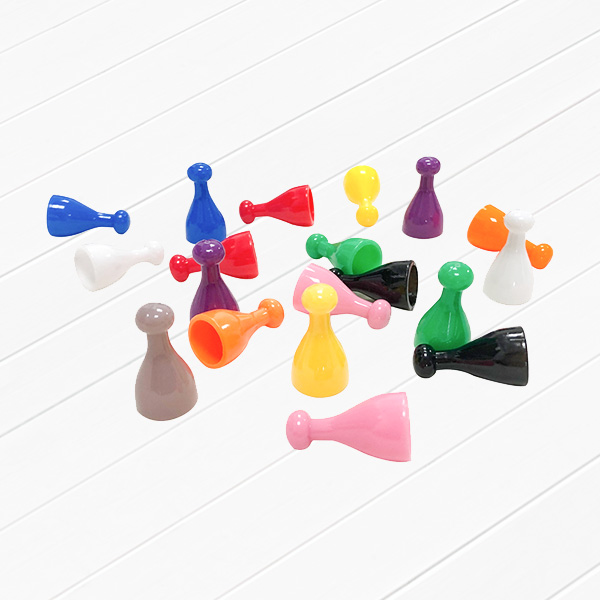This photograph features an assortment of multicolored plastic objects resembling game pieces, likely from a board game such as "Sorry." These pieces are predominantly hollow, shaped like small bowling pins or party hats, with round tops that widen towards the base. The image reveals a vivid array of colors including blue, red, yellow, purple, orange, white, green, pink, gray, and black. Positioned centrally on the off-white, slatted background that might be a table or a leather mat, some pieces stand vertically while others lie horizontally, creating a visually appealing arrangement. The smooth and shiny surfaces of the pieces catch the light, enhancing their colorful appearance. There is no text present in the image.